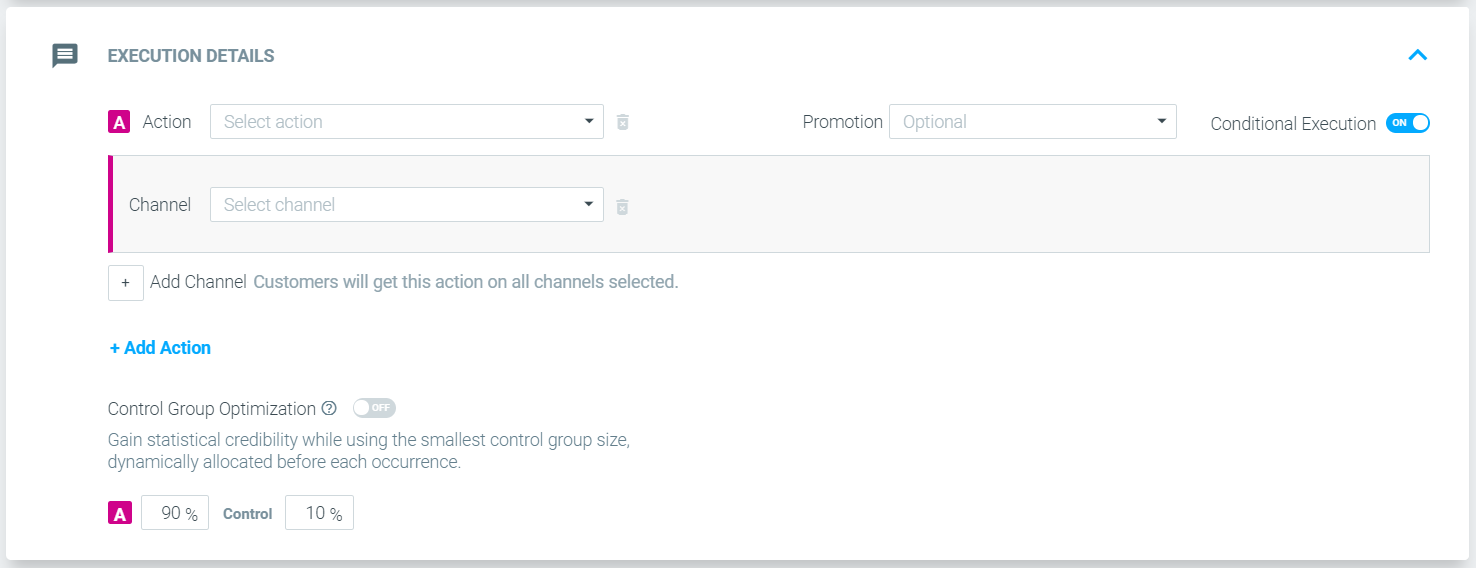A detailed image depicting a web or app interface is shown, framed by a gray border approximately three times as wide and two and a half times as tall. The backdrop is primarily white. In the upper left corner, there is a dark gray speech bubble icon with three horizontal lines, likely a menu option. Adjacent to this icon, bold gray text reads "Execution Details."

Directly below is a white letter "A" within a fuchsia square, followed by the word "Action" next to a drop-down box labeled "Select Action," indicating no selection has been made. Progressing to the right, the text "Promotion" appears about 60% across the image with an adjacent drop-down box labeled "Optional." Further right, "Conditional Execution" is noted with a toggle switch currently turned on.

Returning to the left and moving downwards, a vertical fuchsia bar is visible with the text "Channel" next to a drop-down box, marked "Select Channel," which remains unselected. Beneath this, a white box with a plus sign appears beside the text "Add Channel," indicating actions applicable to all selected channels.

Lower down, a light blue plus sign and the text "Add Action" appear, followed by "Control Group Optimization" in black text. To its right, there is an inactive toggle switch.